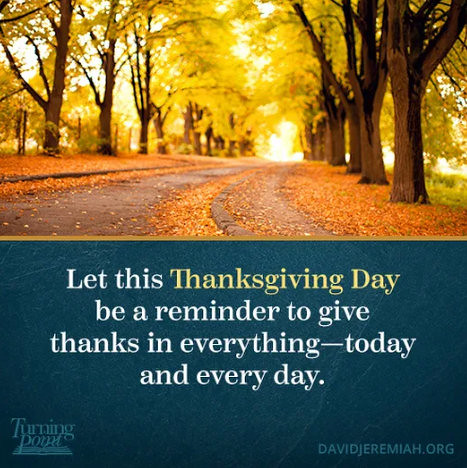The image is a digitally generated graphic poster divided into two sections. The top portion features a picturesque scene of a road or path flanked by large trees with yellow-green leaves bathed in sunlight, creating a golden hue. The road is sprinkled with fallen leaves in shades of orange and yellow, while the center path remains relatively clear. The bottom portion of the poster has a blue background with a quote in white and yellow text: "Let this Thanksgiving Day be a reminder to give thanks in everything today and every day." The bottom left corner features the logo for "Turning Point" with an illustration of an open book, and the bottom right corner displays "DavidJeremiah.org."